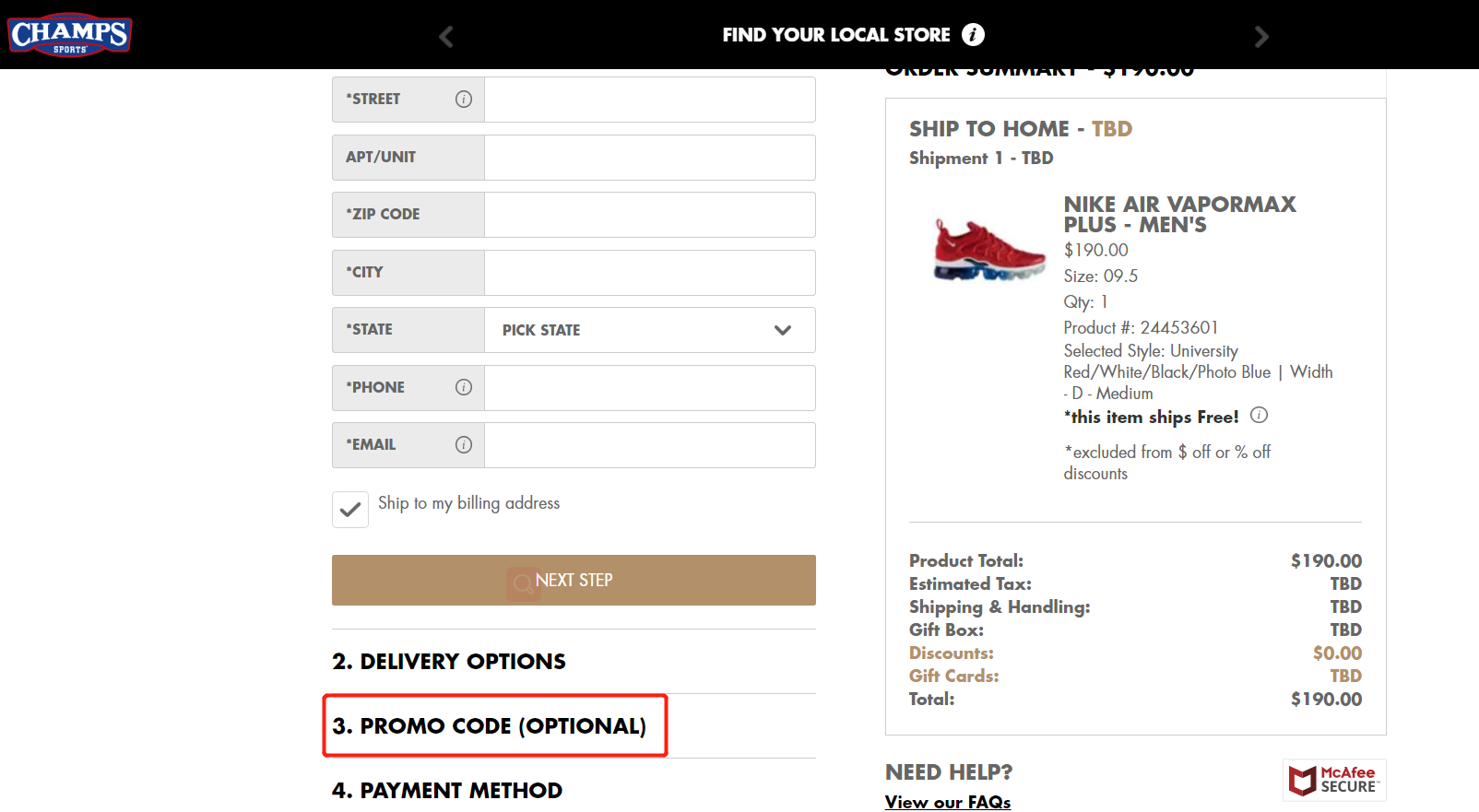This image is a detailed snapshot of a Champs Sports checkout page. At the top, there is an inch-wide black border featuring the Champs Sports logo in the left corner. The logo consists of a blue rectangle with a red border and a semicircle at the top center. In large, bold, white uppercase letters, "CHAMPS" is written across the middle, with "SPORTS" in smaller white letters underneath.

Centered below the logo is the text "FIND YOUR LOCAL STORE" in all-caps bold white letters. Adjacent to this text is a white circle with a black eye icon inside. To the left, about three inches from the top and two inches from the left edge, there are a series of long rectangles. The first third of these rectangles is light blue, transitioning to white for the remaining two-thirds. The first rectangle has black text in its gray section that reads "Street." The subsequent rectangles read "Apartment Unit," "Zip Code," "City," and "State." Only the "State" field has text in the white portion that reads "Pick State." Below this section are fields for "Phone" and "Email". 

There is a checkbox with a black checkmark beside it, labeled "Ship to my billing address." Below this is a large brown button labeled "Next Step" in white text. Underneath, there is a bold number "2" with "DELIVERY OPTIONS" in all-caps, followed by a "3" labeled "PROMO CODE (OPTIONAL)" within a red rectangle border. Next is a "4," labeled "PAYMENT METHOD."

On the right side of the image is the "Order Summary," showing a total of $190. Below this, there are sections labeled "Ship to Home," "TBD Shipment One," and "TBD." To the right, there is a pair of red shoes with details about the shoes, including size and shipping information. A thin line separates this section.

On the left of this line are details labeled "Product Total," "Estimate of Tax," "Shipping and Handling," and "Gift Box," all in black text. Under these, in brown text, are "Discounts" and "Gift Cards," followed by "Total" in black. On the right side, the respective costs are listed. 

At the bottom, the McAfee Security logo is present, and to its left, in bold black text, it says "Need help?" Below this is an underlined text in black that reads "View our FAQs".